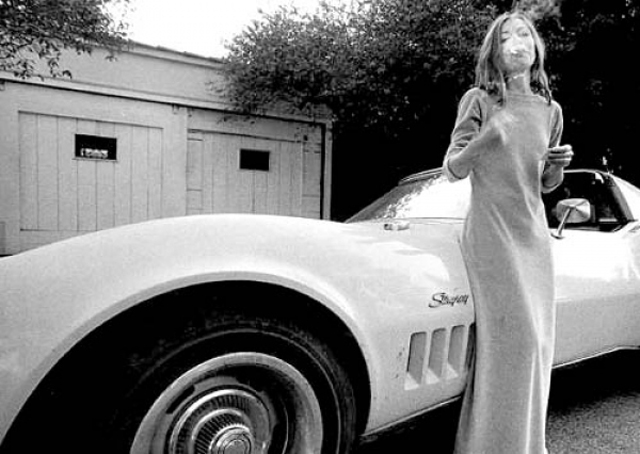This monochrome image captures a young, slender woman wearing a long, foot-length dress with long sleeves, standing in front of a sleek, vintage Corvette Stingray. The car, likely white in color, dominates the center of the frame with its distinctive design, including a large tire and side vents for air. The woman is by the driver's side, leaning against the door, looking directly at the camera. Her shoulder-length hair frames her face, which is veiled in smoke from the cigarette she's smoking, making her features hard to discern. There's a tree in the top left corner and more trees behind the car, indicating a rural setting. To the left of the frame stands a garage or barn with two sliding doors, partially visible under a branch that stretches over its roof. The bright sky reflected off the windshield adds to the detailed capture of this evocative scene.